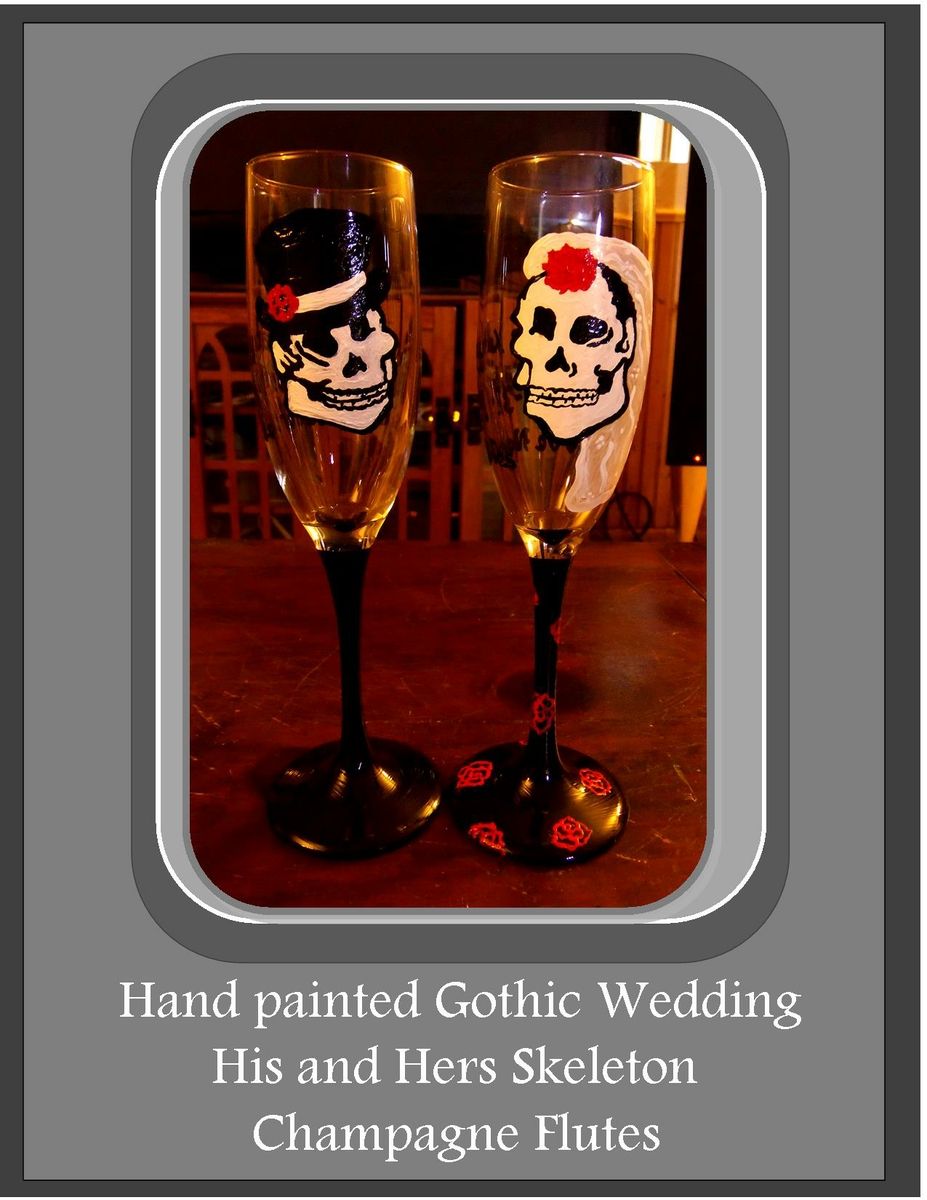This photograph showcases a pair of hand-painted Gothic wedding "His and Hers" skeleton champagne flutes, displayed on a brown table against a nighttime backdrop. Each slender flute features a clear top and a black stem and base. The left flute depicts a skull adorned with a black top hat and a red flower, while the right flute shows a skull with long blonde hair and a red flower at the forehead. The base of the right flute is decorated with red skulls and roses, whereas the left flute has a plain black bottom. The image is framed with a dark and light gray cartoonized plaque frame, which encircles the picture and the white text beneath, which reads "Hand Painted Gothic Wedding His and Hers Skeleton Champagne Flutes." In the background, a gate is faintly visible, adding to the gothic ambiance of the scene.